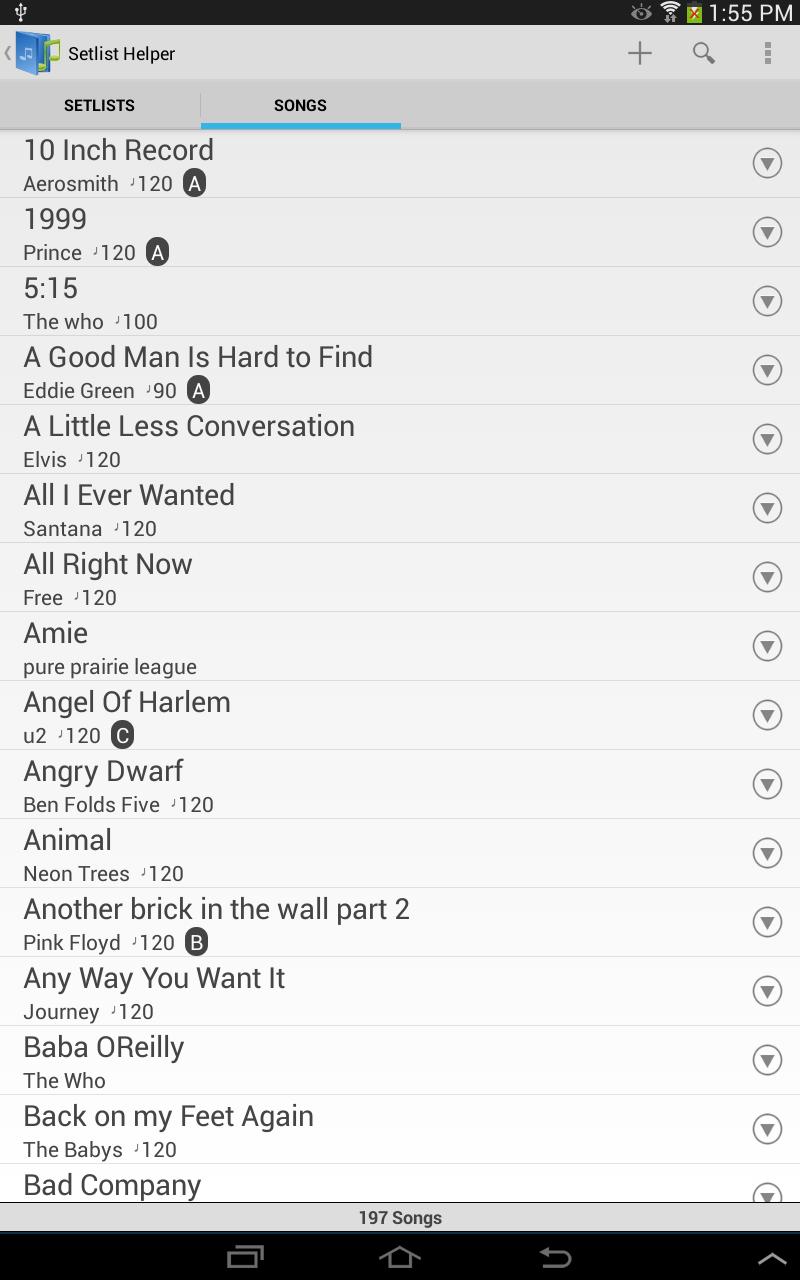This is a detailed screenshot from a smartphone. The top border is black, featuring various icons. On the left side, there's a white icon resembling a candle holder with horizontal extensions. Next to it, the time "1:55 PM" is displayed. A green square with a red "X," a WiFi symbol with two grey arrows beneath, and an eye icon with three eyelashes are all aligned to the right.

Below the black border, the background transitions into a lighter bluish-grey color. On the top left, there's a small blue book icon adorned with a lighter blue music note and a green music note emerging from it. Adjacent to this is the "Set List Helper" label. To the right of the label are icons for a grey plus sign, search functionality, and a vertical ellipsis, all in grey.

A grey border separates these elements from the content below. The top part of this border reads "Set List" on the left and "Songs" on the right, with "Songs" underlined in blue. Listed below are sixteen songs, each separated by thin grey bars. To the right of each song title, there is a grey circle with an upside-down triangle inside.

At the bottom, another thin grey border indicates "197 songs" in black text. Below this, a black border spans the bottom of the screen. Positioned about a third of the way from the left, there's a square icon with a smaller square at its top right corner. To the right, additional icons for home, refresh, and an upward-pointing arrow resembling a greater-than sign are displayed.